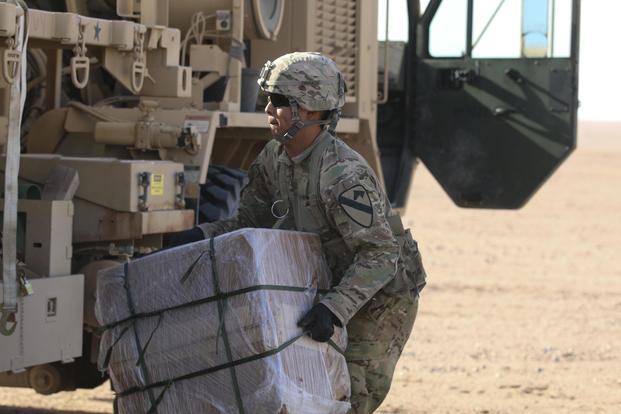In the image, we see a United States soldier operating in an arid desert environment characterized by sandy, dirt-covered ground. The sunlight, which is not directly visible, washes out the upper right-hand corner of the image, creating a bright and stark contrast. The soldier, centrally positioned in the photograph, is dressed in a full camouflage uniform, complete with long-sleeved shirt, pants, black gloves, a strapped camouflage hard hat, and dark sunglasses. 

He is actively loading a package onto a tan or beige military vehicle, which blends seamlessly with the sandy surroundings. The vehicle, akin to a Humvee or other similar military convoy vehicle, is positioned to the soldier's left with its door open at the top. The package in the soldier’s hands is wrapped in plastic and secured with metal straps, obscuring its contents. The scene captures the solitary figure of the soldier in the midst of logistical operations, likely transporting supplies in this remote, sun-drenched desert setting.